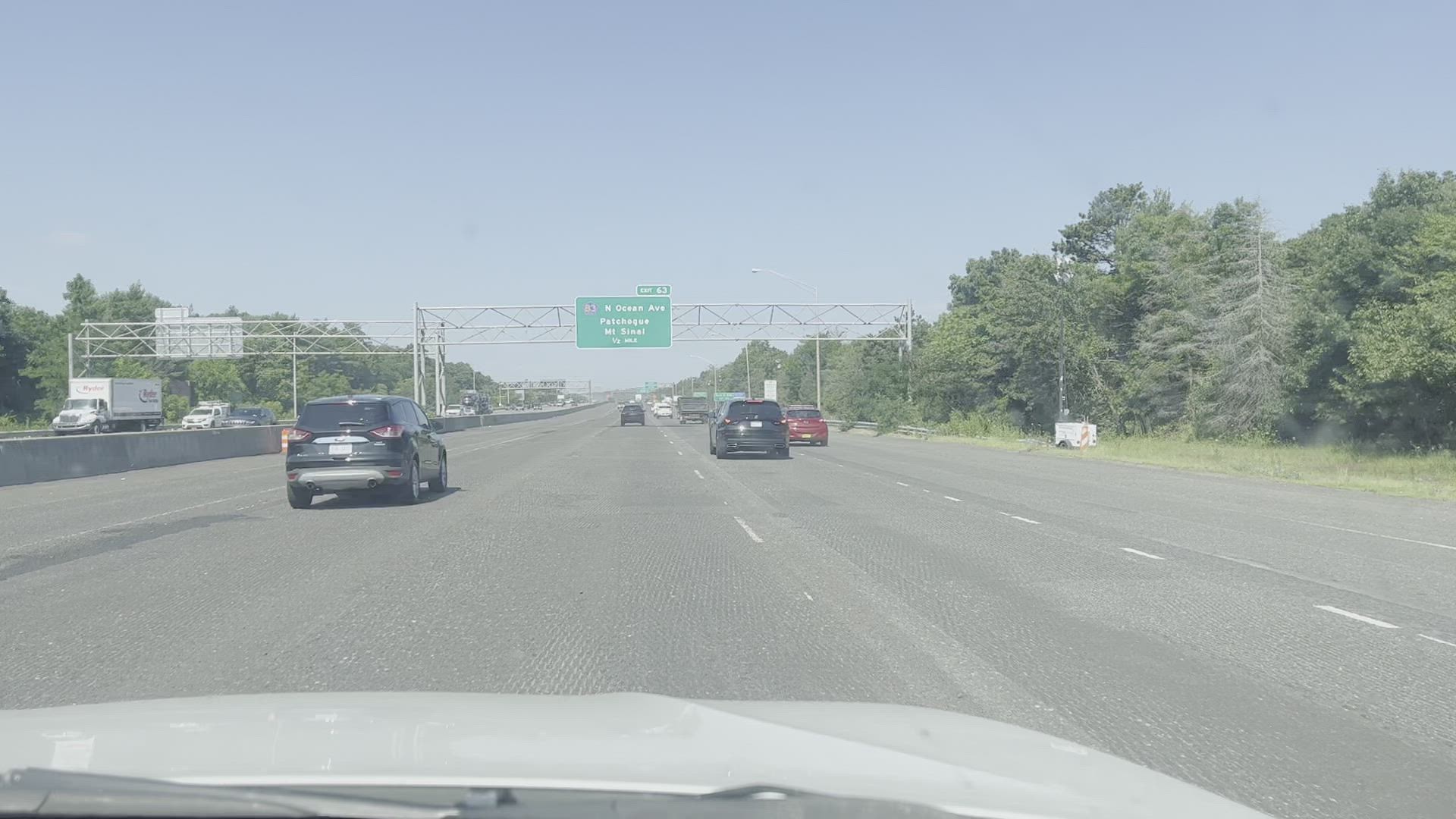The photo captures a highway scene from the front window of a car, with the camera positioned near the windshield, showing part of the car’s hood and a bit of the windshield wiper. The highway consists of five lanes, with some sections suggesting it might stretch to six lanes. In the lane to the left, there is a single car, while the far-left lane appears empty. The roadway ahead is busy with cars in several lanes, including a dark red car approximately six car lengths ahead in the farthest right lane. A large, green directional sign can be seen ahead, but due to a dirty lens, the text is illegible, although it seems to indicate an upcoming exit in approximately half a mile, possibly exit 53. Further details suggest the exit could be North Green Avenue, which would be exit 63. The image is clear enough to show a blue, cloudless sky and dense foliage of various heights lining both sides of the highway. A concrete barrier separates the oncoming traffic on the left from the lanes depicted. Additional roadside details include something that seems like a temporary sign stand and an abandoned box resting on the berm to the right.